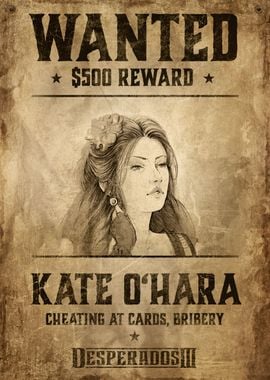This image depicts a vintage-style wanted poster, evocative of the old American West, but created in the modern era. The background mimics aged, weathered brown paper. At the very top, large dark brown letters declare "WANTED," followed by "$500 REWARD" in a smaller, yet equally dark font. Below this, a black and white illustration of a woman occupies the center of the poster. The woman, likely in her twenties or thirties, is depicted with long brunette hair, styled with a braid on one side, adorned with a flower clip, and wearing earrings. Underneath the illustration, the name "KATE O'HARA" is prominently displayed in dark brown letters, succeeded by the accusations: "CHEATING AT CARDS" and "BRIBERY." The bottom of the poster features the title "DESPERADOS 3," suggesting that this image is associated with a film or video game series of the same name. Two small black stars flank the text, reinforcing the vintage aesthetic.